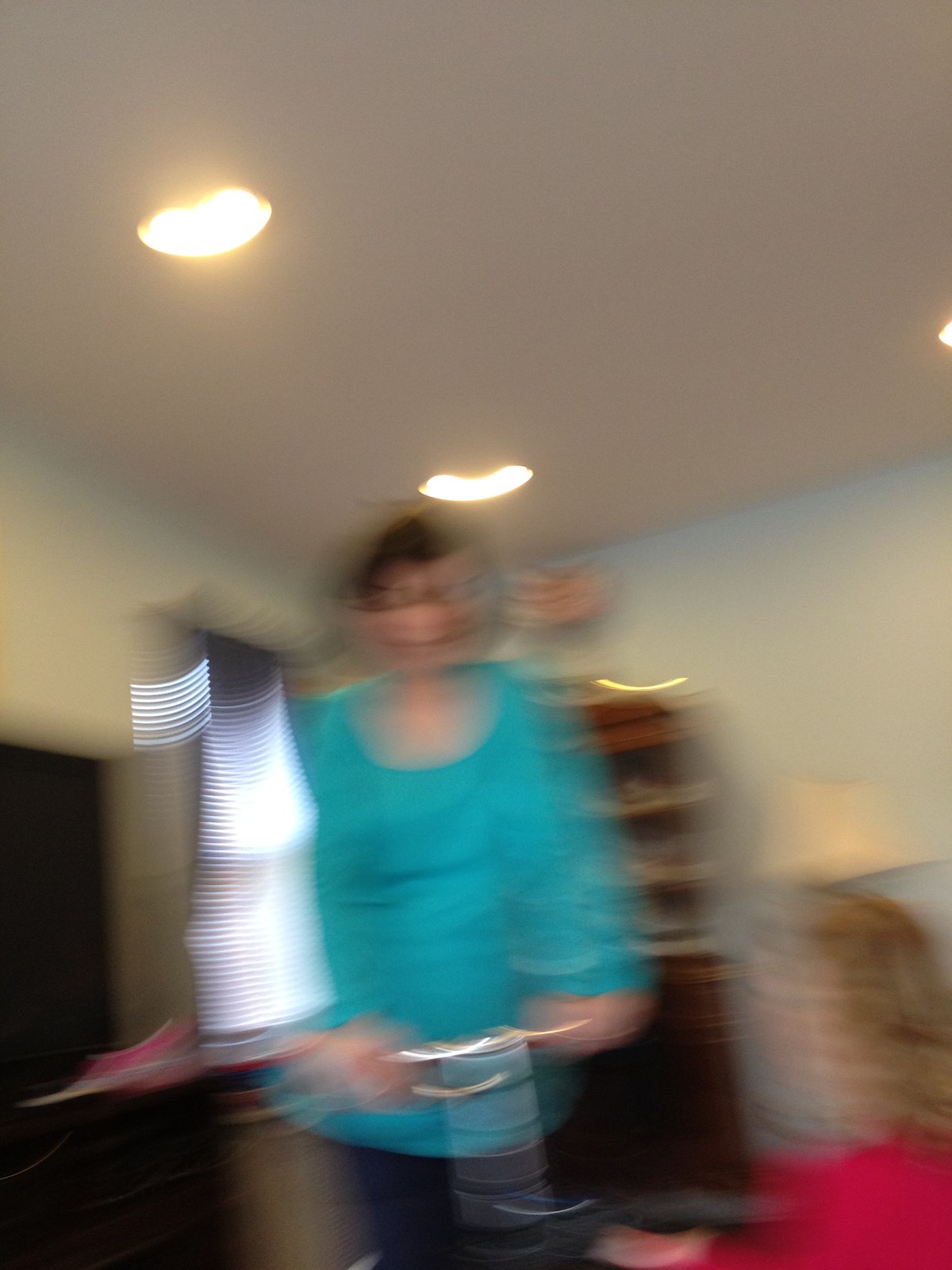A very blurry, motion-distorted photograph shows a scene inside a living room. In the image, a Caucasian woman appears to be standing with a teal-colored, long-sleeve blouse and dark pants. She has short brown hair, possibly smiling, and her hands seem to be clasping something, perhaps a plate. In front of her, there is another Caucasian woman with long, dirty blonde hair, wearing a long-sleeve red top, seated. The photo captures a first-person perspective, suggesting the photographer is sitting down, with the camera at waist level to the standing woman. The background features a wooden shelf or cabinet, a TV, a window with blinds partly open allowing sunlight to filter through, and a flat ceiling with built-in lights.